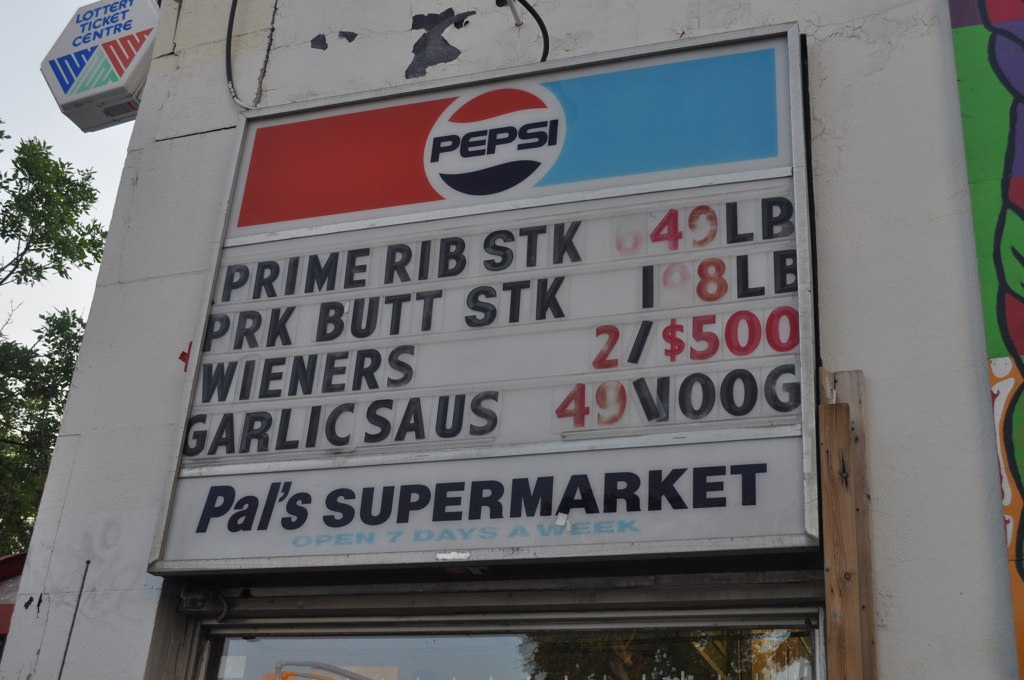A weathered outdoor sign stands outside Pal's Supermarket, open seven days a week. The sign displays the vintage Pepsi logo at the top, adding a nostalgic touch. Below, plastic slots allow for customizable messages. At the top of the sign, a blue banner with red and silver or green accents, and squiggly lines, proudly announces "Lottery Ticket Center," although it's noticeably faded from prolonged sun exposure.

Pal's Supermarket has chosen to advertise the following deals in four distinct lines:

1. Prime Rib Steak (abbreviated as STK) at $6.49 per pound.
2. Pork Butt Steak (abbreviated as PRK, butt with two 'T's, and STK) at $1.98 per pound.
3. Wieners at two for $5, likely referring to two packets.
4. Garlic Sausage (abbreviated as SAUS) at $0.49 per 100 grams, suggesting the location could be in Europe due to the metric measurement.

The sign, with its mix of faded colors and time-worn appearance, speaks to the enduring legacy of Pal's Supermarket in the community.